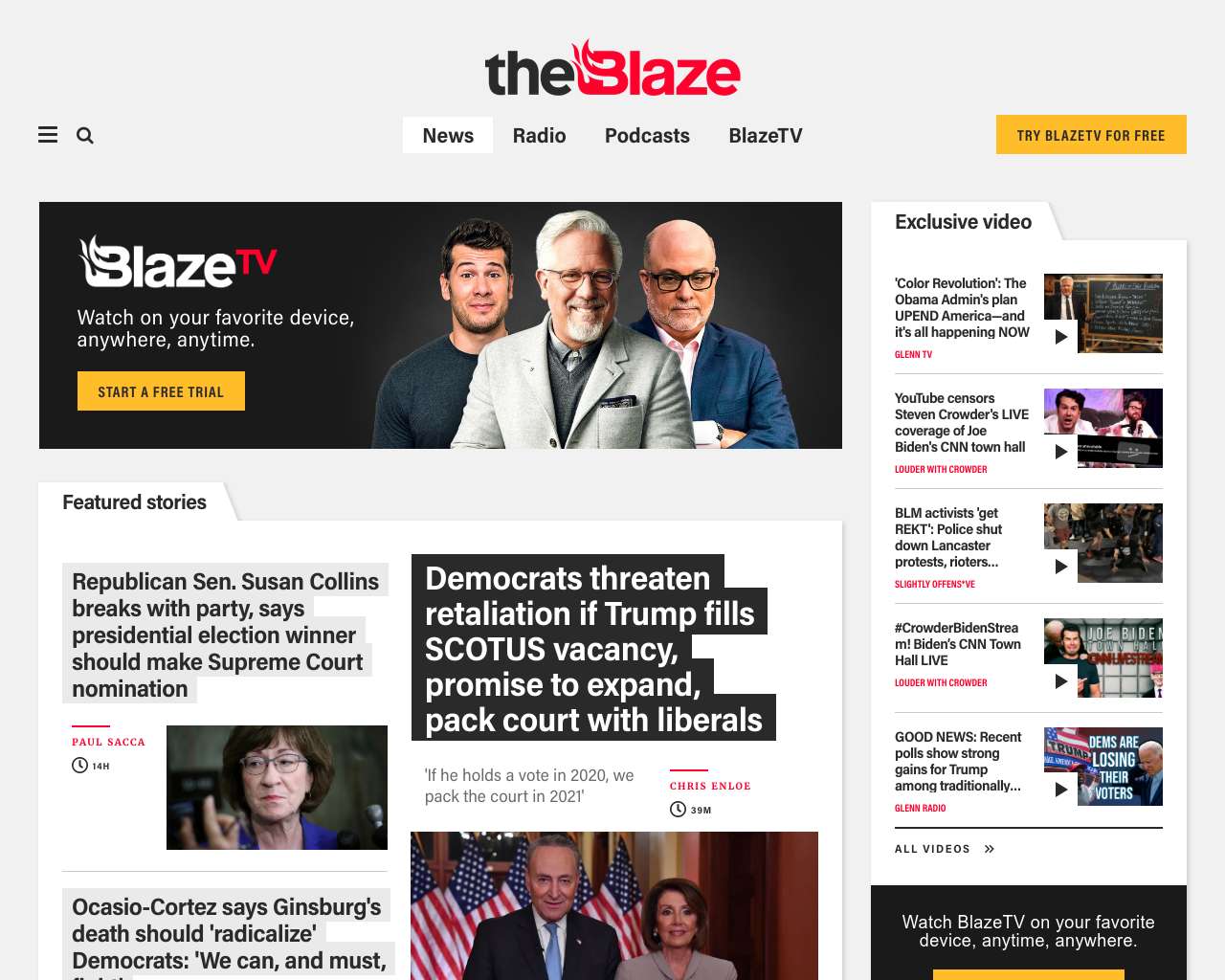This image is a detailed screenshot of The Blaze, an online news site founded by Glenn Beck. The background is a light gray, creating a minimalistic, clean aesthetic. Centered at the top is the logo: "The Blaze" with "The" in bold black lowercase letters and "Blaze" in red, initial-capped letters. The "B" in "Blaze" is stylized with flames extending from the left side.

Directly beneath the logo is the menu bar, featuring categories in black font: News, Radio, Podcasts, and Blaze TV. On the right side of the menu is a gold rectangle with an invitation in black text to "Try Blaze TV for free."

The main section of the page features a large dark gray rectangle showcasing three prominent figures: Glenn Beck, Stephen Crowder, and Mark Levin. Glenn Beck, with silver-gray hair and a matching mustache, is dressed in a gray suit jacket. Stephen Crowder is seen in a long-sleeve black t-shirt, sporting brown hair and a hint of a beard. Mark Levin, bald and wearing black-framed glasses, is clad in a medium-blue suit jacket. Each of these individuals is a white male, and their photos are displayed prominently.

To the left of these images, "Blaze TV" is written in white on a black background, with "TV" in a smaller red font. Below this, it reads: "Watch on your favorite device, anywhere, anytime," followed by another gold rectangle stating "Start a free trial."

Scrolling further down, a collection of headlines and stories is visible. The left headline reads: "Republican Senator Susan Collins breaks with party, says presidential election winner should make Supreme Court nomination." To the right, another headline in white text against a black background announces: "Democrats threaten retaliation if Trump fills SCOTUS vacancy, promise to expand PAC court with liberals."

Additionally, on the right sidebar labeled "exclusive videos," more stories and headlines are presented, curating a comprehensive glance at the latest news.